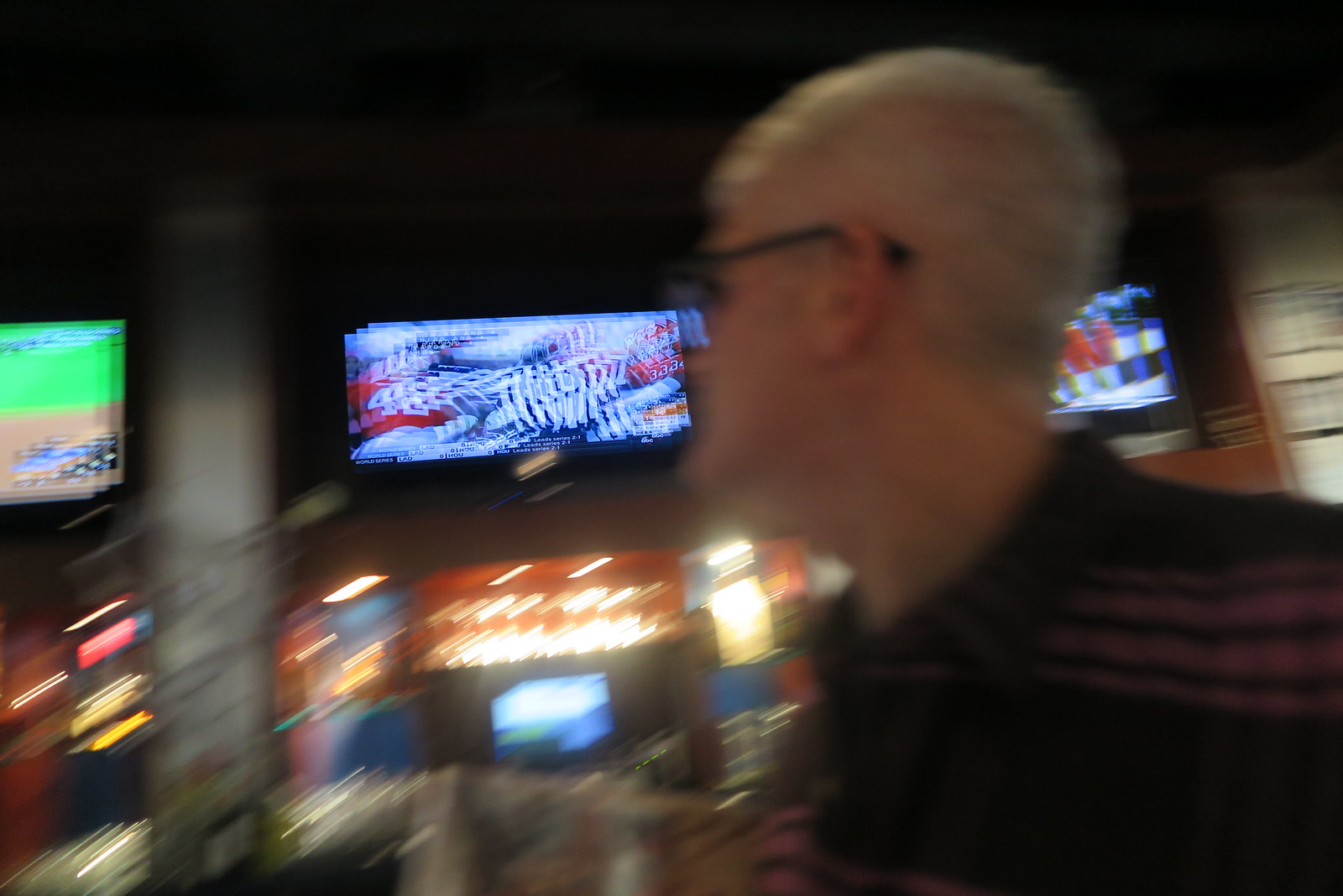In this blurry, low-light indoor image (landscape aspect ratio), a human male is visible on the right side, captured in profile view from the face to the upper torso. He sports grayish-white hair, black glasses, and has a light skin tone. The left side of the image is dominated by motion blur, suggesting the camera was moved rapidly at a slow shutter speed, resulting in dynamic light streaks across the room. Above, three televisions are partially discernible; the left screen seems to display a baseball diamond, likely from a baseball game, the middle screen appears to feature an NFL football game, while the content of the right screen remains unclear. The combination of these details implies that the setting is possibly a sports bar or a hotel lounge.